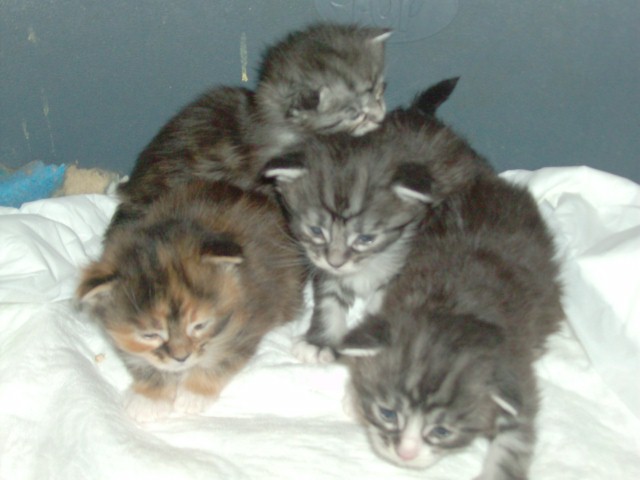In this somewhat blurry and low-quality yet adorable photo, four fuzzy kittens are nestled closely together on a white duvet or comforter, likely on a bed. Behind the kittens, the walls are painted a bluish-gray color. Three of the kittens have gray and white fur with blue eyes, showcasing pale gray coats with darker gray stripes, while the fourth kitten, positioned on the left, is a calico with orange and black fur, its eyes downcast and not clearly visible. The three gray kittens lie side-by-side, with the central one appearing to prepare to stand. The fourth, smaller gray kitten is perched atop the middle gray kitten, its head resting on the others' back and looking off into the distance at the bottom right of the frame. This cozy arrangement highlights the kittens' semi to medium-long fur and their endearing demeanor.